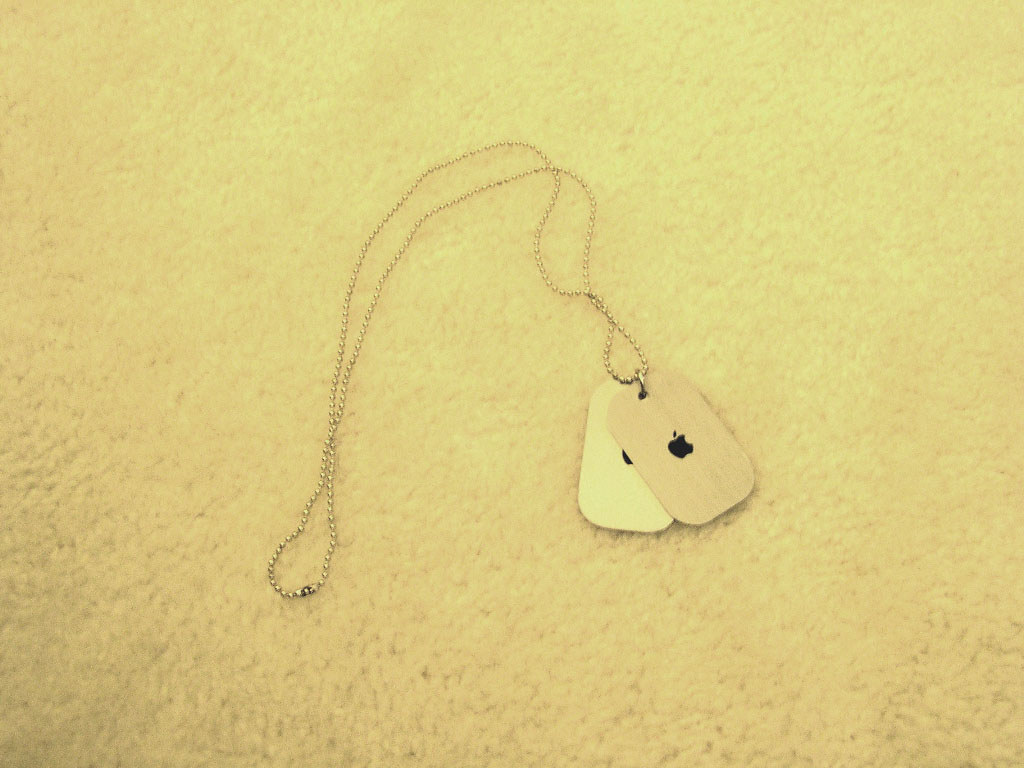The photograph captures a necklace styled like military dog tags, with two rectangular cardboard tags, each displaying the iconic black Apple logo with the bite taken out. The chain is made of beaded metal and is positioned centrally, trailing toward the bottom of the image. The two tags are of different shades—one light brown and the other white—yet both bear the same Apple insignia. The necklace rests on a cream-colored shag carpet, creating a yellowish-white, neutral undertone across the frame. The overall image appears slightly blurry with some areas looking more grayish, especially toward the lower left corner, emphasizing the monochromatic and subdued palette of the scene.